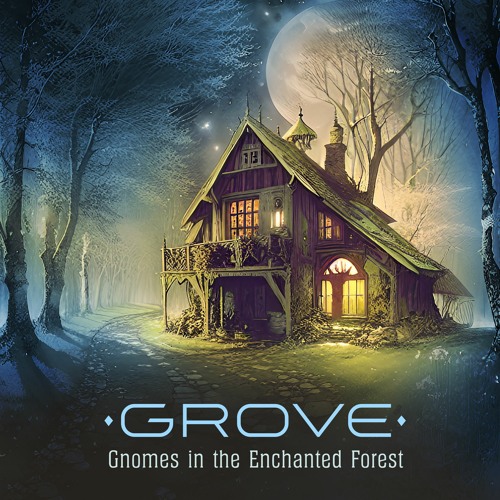This detailed digital artwork features a cottage-style house centrally located within a snow-covered forest, giving the piece a fantasy ambiance. The house, which stands as a two-story structure with a single large roof, is adorned with glowing yellowish lights emanating from its windows and glass front doors. A pathway leads to and circles around the cottage, with the surrounding grass tinged green under the illuminated windows, contrasting sharply against the prevalent white, possibly indicative of snow or moonlight.

The forest is dense with tall trees, their white leaves hinting at either snowfall or the reflective effect of a large, bright moon looming above in the night sky, partially obscured by the canopy behind the house. The scene feels eerie, with an overarching blue and orange haze adding to its mystical atmosphere. A fog or haze envelops the background at the base of the image, enhancing the enchanting, otherworldly feeling. Vines grow around the cottage doors, and there's a balcony aligning with a second-floor door, alongside a chimney atop the roof.

Prominent at the bottom of the image, large light blue text reads "GROVE," with smaller white text underneath spelling out "Gnomes in the Enchanted Forest," suggesting a magical or fantastical storyline, akin to a book cover illustration.